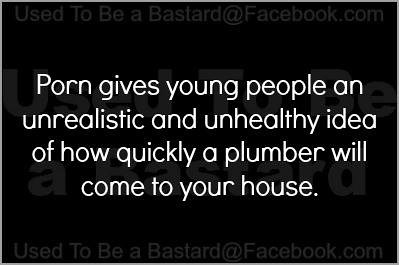This is an image of a Facebook post against a completely black background with centrally positioned text. The main feature of the image is a message displayed in slightly uncrisp, white, thin lettering that reads: "Porn gives young people an unrealistic and unhealthy idea of how quickly a plumber will come to your house." The text is divided into four rows and ends with a period. At the top of the image, barely visible, there is a light green shadow obscuring what seems to be an old web address ending in "book.com," blending almost imperceptibly into the dark background. The entire presentation lacks any additional images or icons, focusing solely on this singular, bold statement.